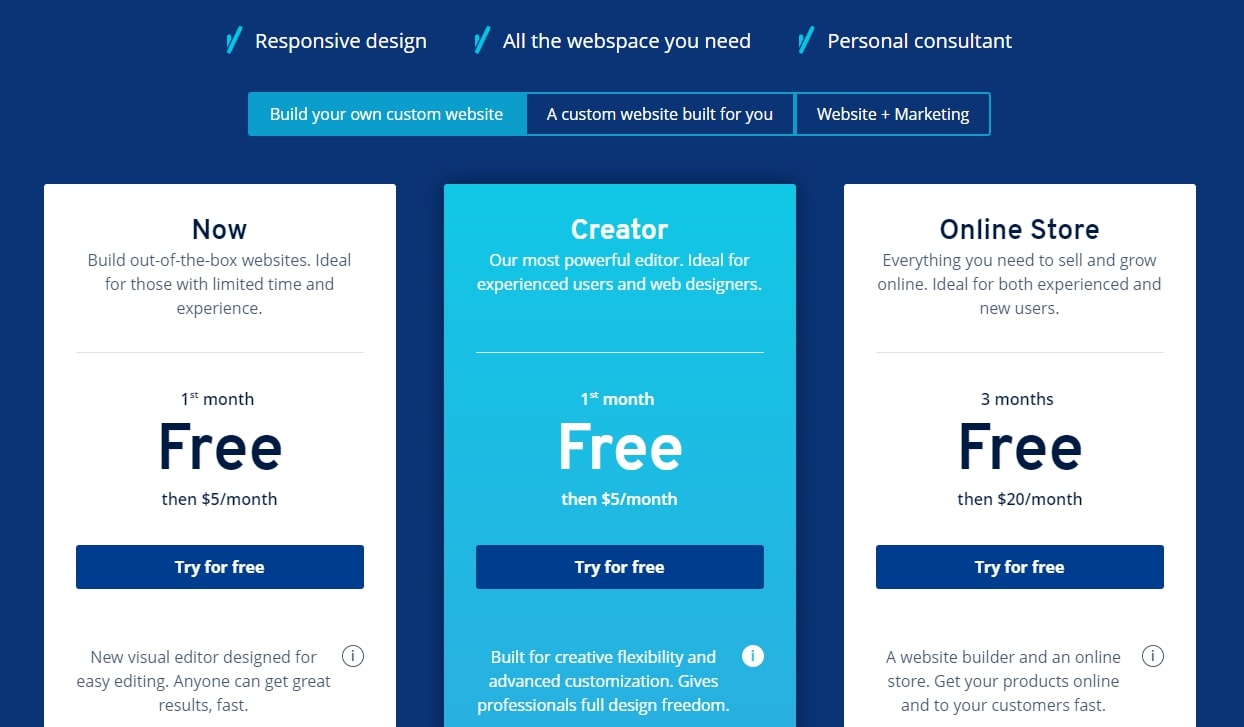The image depicts a blue-themed web page dedicated to website creation services. At the top, three key features are highlighted in white text next to blue checkmarks: "Responsive Design," "All the Web Space You Need," and "Personal Consultant."

Below these features, three boxes offer detailed service options:

1. The first box, with a light blue background, is labeled "Build Your Own Custom Website." This option is designed for users with limited time and experience, offering out-of-the-box websites. The first month is free, followed by a $5 per month subscription. Additionally, it features a blue "Try for Free" button and mentions a new visual editor made for easy editing, ensuring that anyone can achieve great results quickly.

2. The second box, in a deeper blue hue, is titled "Creator" and is described as their most powerful editor, ideal for experienced users and web designers. This option also offers the first month free, then costs $5 per month. It features a blue "Try for Free" button and highlights its capability for creative flexibility and advanced customization, providing professionals with full design freedom.

3. The third box, focused on e-commerce, is labeled "Online Store." It claims to have everything needed to sell and grow online, suitable for both experienced and novice users. The service is free for the first three months and then costs $20 per month. A blue "Try for Free" button is located here as well, and the service is described as a website builder combined with an online store, facilitating quick product listings and customer reach. 

Additionally, each box comes with descriptive tags and benefits to help users decide the best plan based on their needs and expertise.